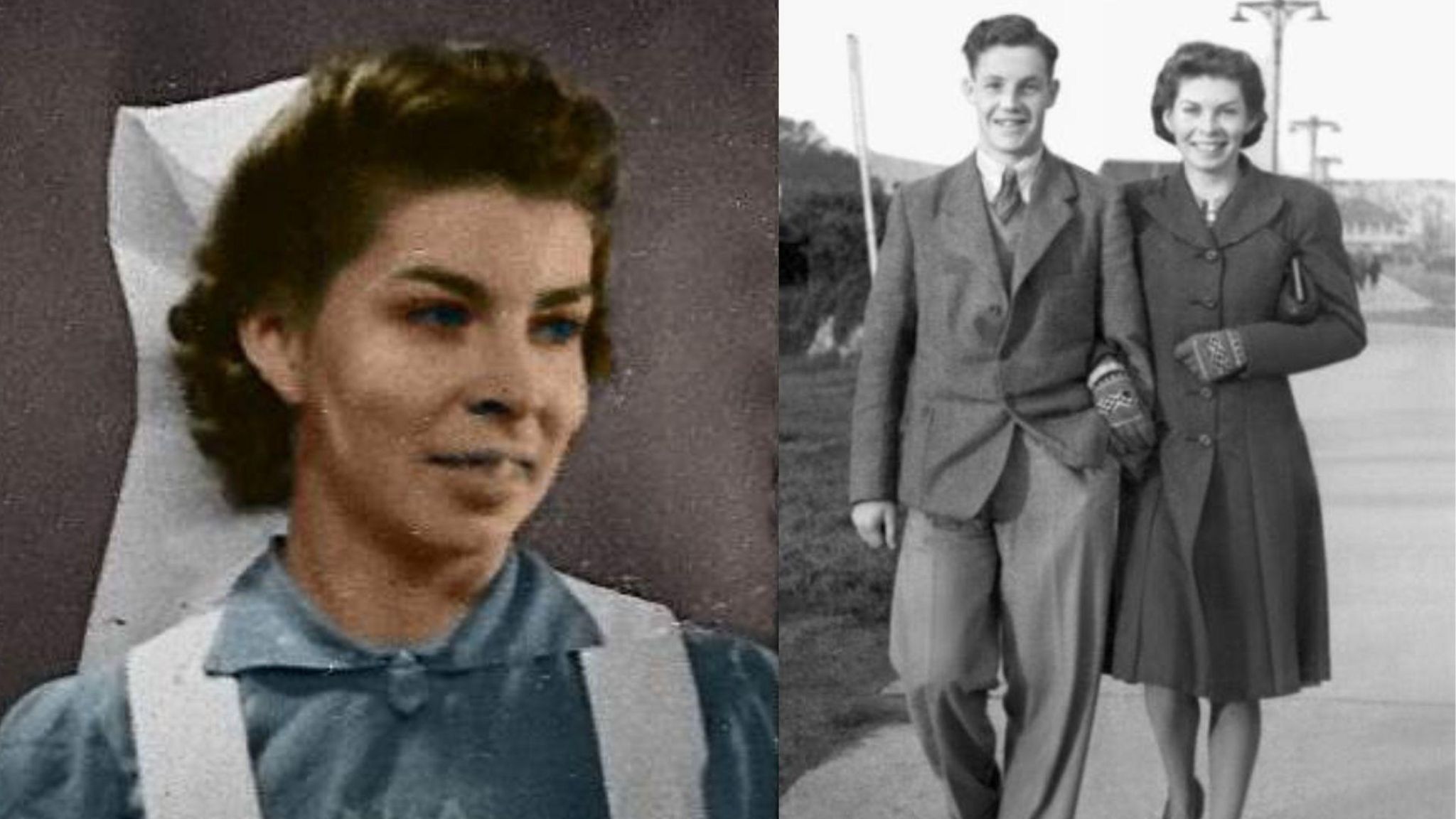The image consists of two vintage, black-and-white photographs placed side by side to form a single, continuous scene. The left photograph, which has been colorized, features a close-up portrait of a white woman in her late 20s or early 30s dressed in a nursing uniform. She has short, dark, curly hair, blue eyes, and is wearing a white nursing cap that drapes behind her head and a teal blue blouse buttoned up at the neck, accented with white straps. She is looking to her right with a gentle smile on her face. Set against a gray background, this photograph exudes a nostalgic 1950s ambiance.

The right photograph remains in its original black-and-white format and depicts the same woman walking down a street, arm-in-arm with a man dressed in a gray suit and tie. She has donned a fancier dark gray blazer and gloves, with her left arm crossing her chest. They both smile warmly and look upwards as they walk along a sidewalk, with power lines and streetlights faintly visible in the background. This juxtaposition of images, one colorized and one in classic black-and-white, beautifully captures a moment in time, blending close-up intimacy with an outdoor narrative of companionship.